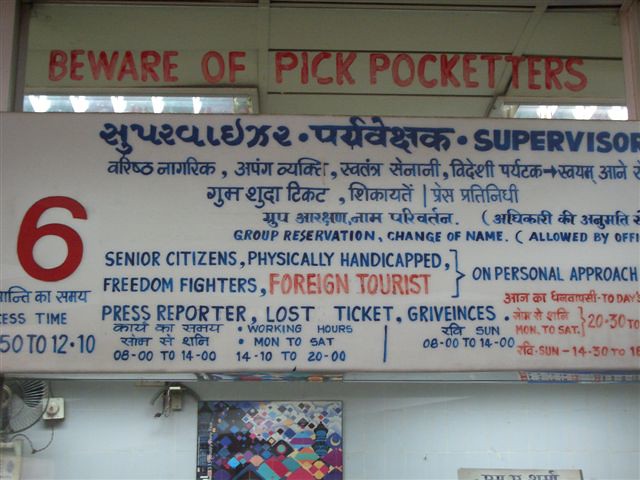In this image, a prominently displayed warning at the top reads "Beware of pickpocketers" in bold red letters painted directly onto a white wall. Below this warning, a long rectangular sign, positioned vertically, features text in both a foreign language and English. The top half of the sign is mostly in blue and includes the word "Supervisor" in bold font. Moving down the sign, the English text begins with "Group reservation, change of name, allowed by office" and continues with listings for "Senior citizens, physically handicapped, freedom fighters, foreign tourists," all of which require a personal approach. Additional information on "lost tickets or grievances" is also provided. 

In a striking red color, a large number six is situated on the left side of the sign. At the bottom of the sign, working hours are specified as "Monday to Saturday, 1410 to 2000." The setting around this sign includes a silver fan attached to the wall on the bottom left side, and below the sign, a multicolored geometric artwork is visible against the light blue wall. On the bottom right-hand side, there is an additional white sign, though its text is unreadable.